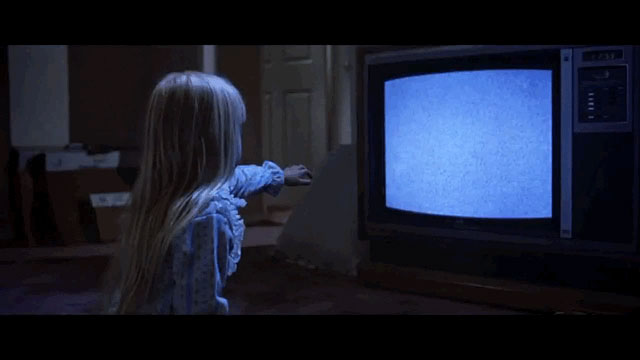The image, seemingly a still from the movie "Poltergeist," exudes an eerie atmosphere, predominantly dark except for the ghostly glow emanating from the TV screen engulfed in static. At the center of the scene is a young blonde girl, likely the famous child actress who tragically passed away after the film's release. She is enrobed in blue and white pajamas or a dress, her long, straight blonde hair flowing as she sits facing the TV. The room's lights are off, accentuating the contrast between the inky darkness and the TV's flickering light that illuminates the girl's figure. She is reaching out with her left hand towards the TV, adding to the haunting ambiance. Behind her, the background reveals an open doorway leading into a hallway, with some indistinct white squares and piled-up boxes barely visible in the murky shadow. The TV itself, old-fashioned with a silver border and a control panel on the right, is the focal point of her attention, casting an otherworldly light upon the scene.